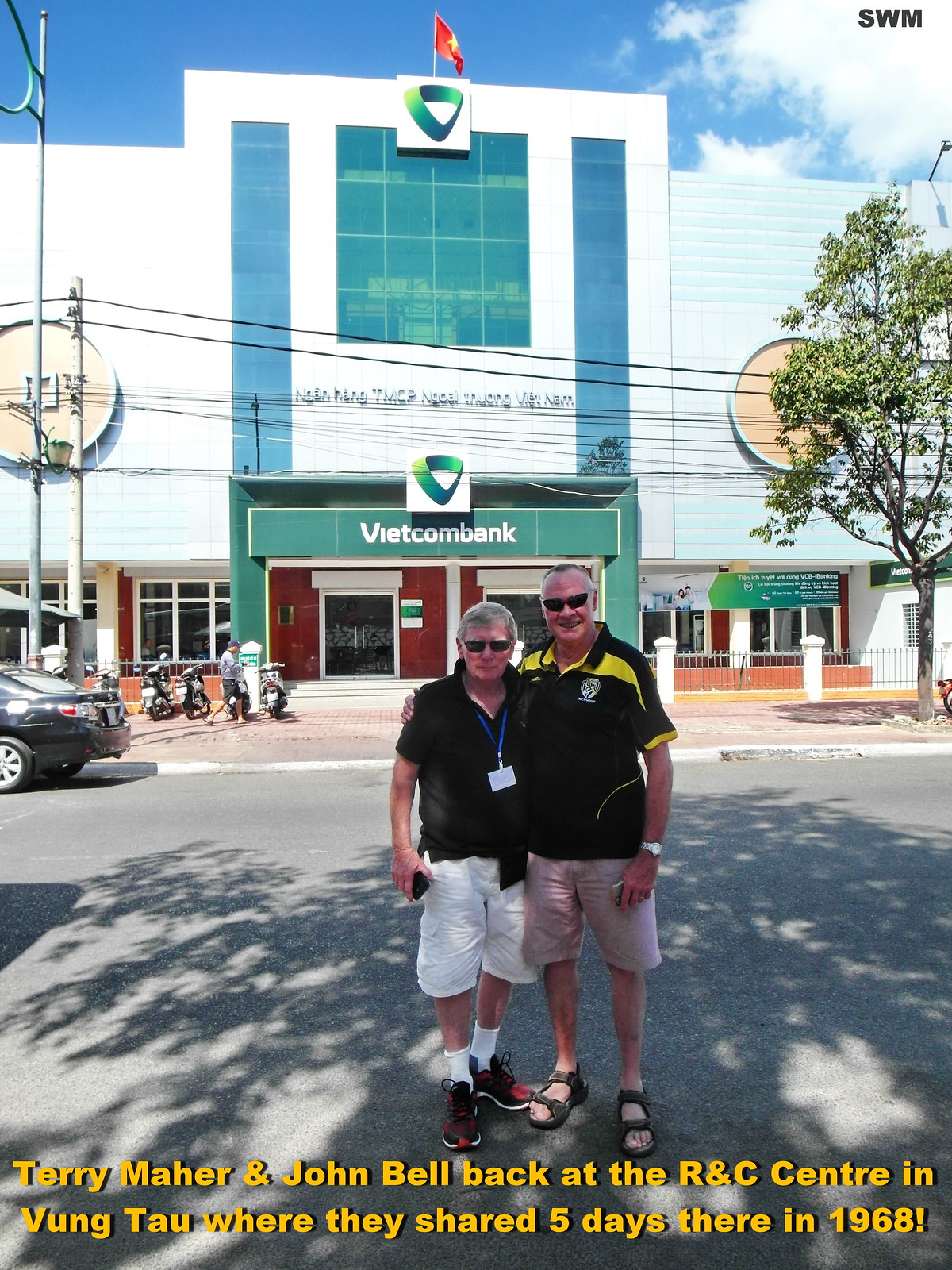In this color photograph with portrait orientation, two older Caucasian men are smiling and posing for the camera in front of a two-story white building with green accents and bluish windows, labeled Vietcom Bank. Both men, who have gray hair and are wearing black sunglasses, have their arms around each other’s shoulders. They are dressed in short-sleeved black polo shirts, with the taller man on the right also sporting yellow accents on his shirt. The man on the left is wearing white shorts, socks, sneakers, and holding a smartphone, while the man on the right is in light pink beige shorts and open-toed sandals. The backdrop features a Vietnamese flag with a red background and a yellow star, a cluster of motorcycles, and a parked car. Typed in yellow at the bottom of the image are the words: "Terry Maher and John Bell back at the RNC Center in Vung Tau, where they shared five days there in 1968." The photograph captures a moment of camaraderie and nostalgia against a historically rich urban setting.